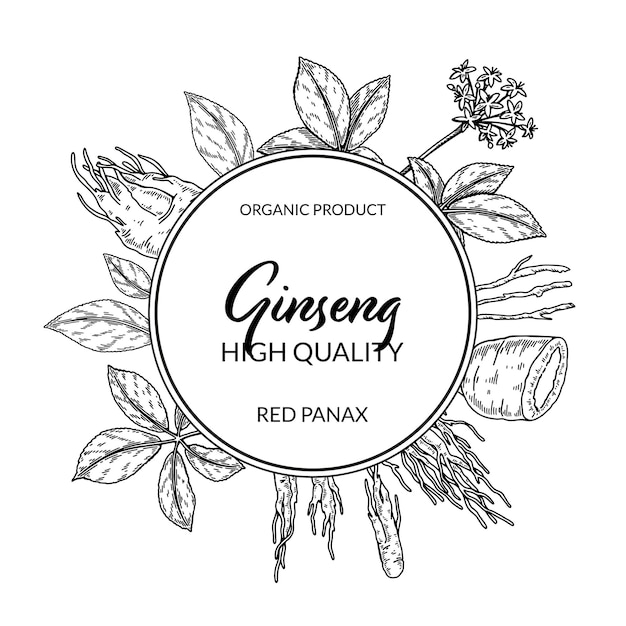This is a detailed black and white digital pen drawing, representing a label for an organic ginseng product. At the center of the image is a circular design bordered by two thin concentric lines, one black and the other lighter in shade. Inside the circle, the phrase "organic product" is written in small, centered capital letters. Below this, the word "ginseng" appears in a script font, followed by the larger, uppercase text "HIGH QUALITY." Beneath this, the smaller capital letters spell out "RED PANAX."

Surrounding the central circle is a rich, intricate array of different types of leaves and flowers. On the top right, there is a stalk adorned with little flowers, while the rest of the circle is flanked predominantly by varying clusters of leaves. These clusters include groups of three to five leaves, and contribute to the detailed and natural frame of the design. The entire composition integrates these botanical elements seamlessly into the overall aesthetic of the label, providing an elegant and organic look.